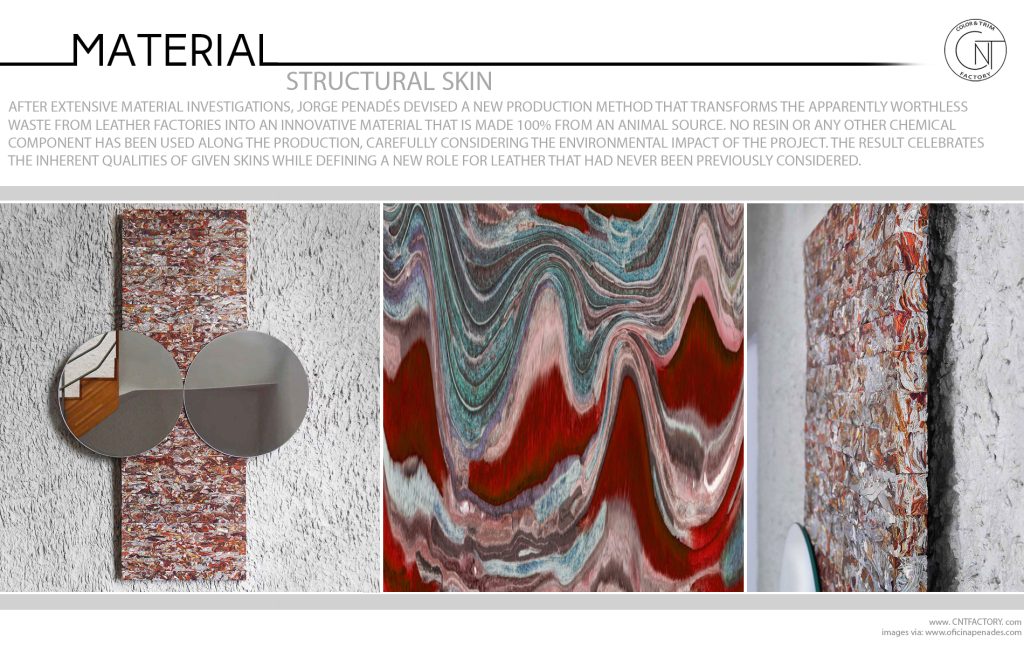This image presents an informational brochure titled "Material" in bold, black uppercase letters at the top, followed by the label "Structural Skin" in gray. The central paragraph describes how George Pinedas developed an innovative production method that transforms waste from leather factories into a 100% animal-source material, devoid of resin or chemical components. Emphasizing environmental mindfulness, the process showcases the intrinsic qualities of leather, redefining its use in unprecedented ways.

The image includes a horizontal arrangement of three photographs beneath the textual description. The left photograph depicts a long, rectangular piece with two overlaying gray circles, reminiscent of an abstract design or an artwork made from the new material. The middle photograph offers an up-close view of the intricate texture, revealing an array of smeared colors such as red, blue, green, black, and gray. The right photograph provides another close view, showing the artwork displayed against a black and white wall, highlighting the detailed and vibrant nature of the material.